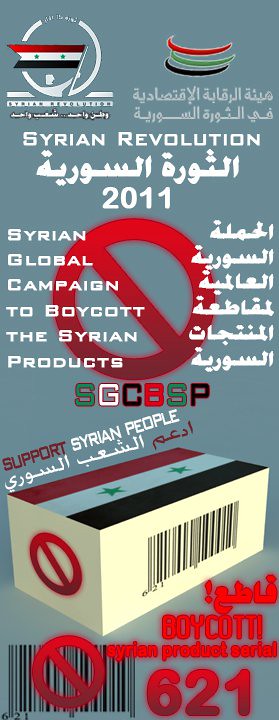The advertisement, vertically oriented with a pale blue background, advocates for the boycott of Syrian products. Featured prominently at the top, the ad showcases symbols including the Syrian flag, characterized by three horizontal stripes—red, white, and black—with two green stars. Beside the flag is another icon resembling a swirl with colors transitioning from red to light green, and then to dark green or black. The text "Syrian Revolution 2011" is displayed in English, paired with words in another language, presumably Arabic. Below this, in large white text overlaying a red circle with a diagonal line (a universal symbol for prohibition), the text reads "Syrian Global Campaign to Boycott the Syrian Products" and the acronym "S-G-C-B-S-P" followed by "Support Syrian People". Further down, a white box-like imagery features the Syrian flag and a prominent barcode on the front. Flanking the box is another circled prohibition symbol. Below the box, the words "Boycott Syrian Products" appear in red letters alongside the serial number 621, and yet another barcode at the bottom left corner, marked by a red prohibition sign.